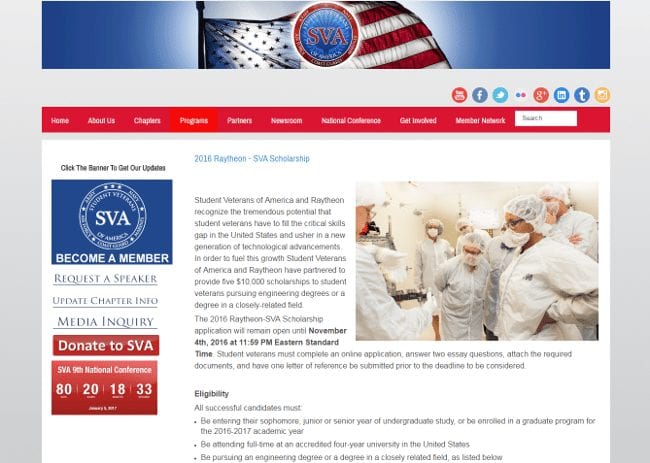The website features the logo of the Student Veterans of America (SVA) prominently at the top. The logo consists of a circular emblem with a blue center, a red "SVA" inscribed in the middle, and additional text encircling it, though the outer text is difficult to discern. The background of the page includes a photograph of the American flag, with light illuminating the blue field and stars, framed by a clear blue sky on either side.

Below the main header, there's a red navigation bar with white text, offering links to sections such as "Home," "About Us," "Chapters," "Programs," "Partners," "Newsroom," "National Conference," "Get Involved," and a partially readable section that likely includes the term "Network." This bar also features a white search box. 

To the right of the search bar, there are social media icons for Facebook, Twitter, Google+, Instagram, and possibly Tumblr. 

A banner below these elements invites visitors to "click the banner to get our updates." On the left side of the screen, there are several actionable links: "SVA," "Become a Member," "Request a Speaker," "Update Chapter Info," "Media Inquiry," and "Donate to SVA." Additionally, there is a promotion for "SVA's 9th National Conference," likely including dates and times, though the specific details are unreadable. 

Lastly, the banner mentions the "2016 Raytheon SVA Scholarship."